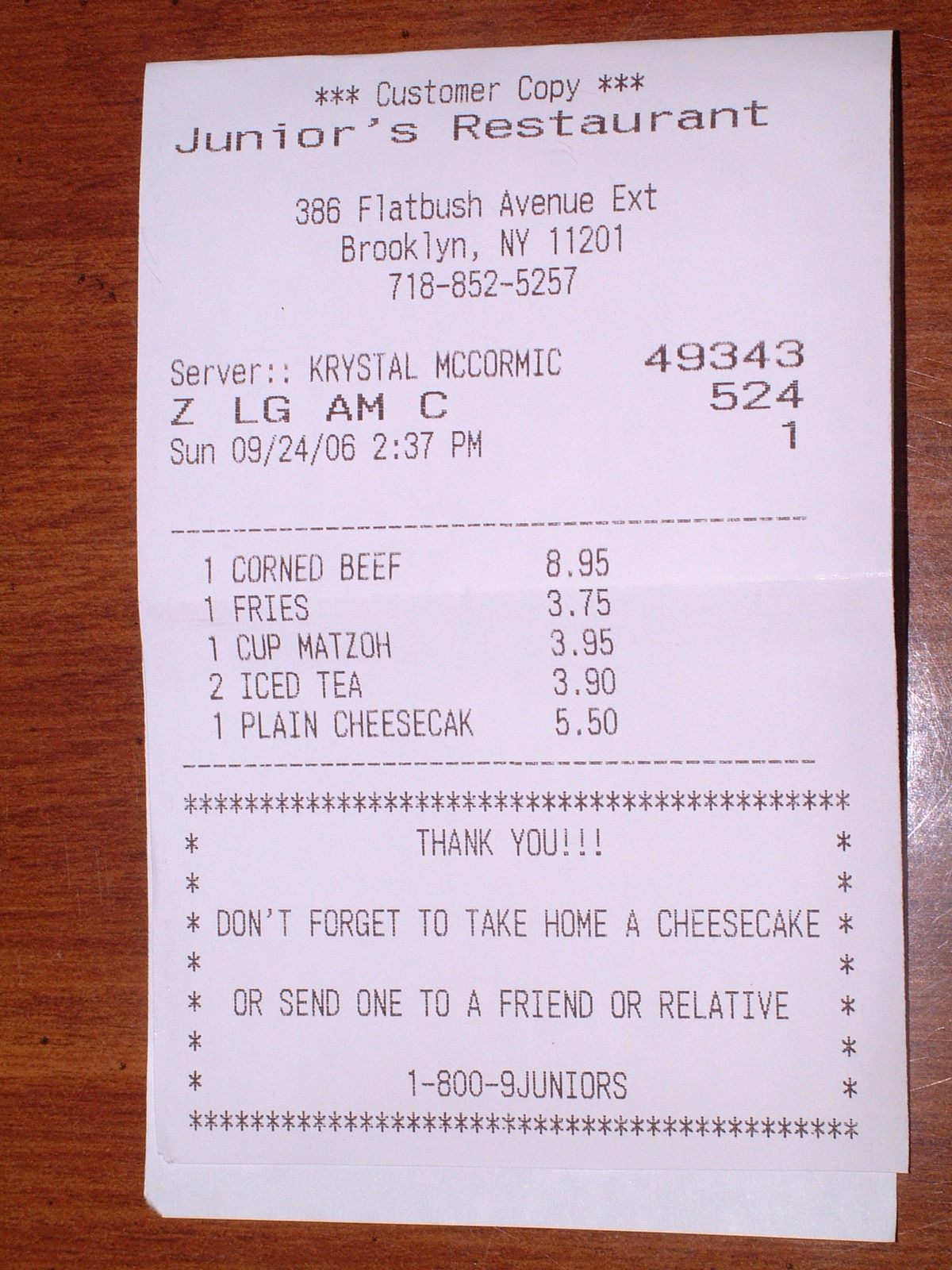This is a close-up photograph of a short receipt printed on white paper with black ink. At the top of the receipt, centered and flanked by three asterisks on each side, are the words "Customer Coffee." Directly below, in larger text, is the name "Junior's Restaurant," followed by the restaurant's address and phone number. The receipt details the server's name, "Crystal McCormick," and includes her server number. A dashed dividing line separates the header from the itemized list of ordered foods and beverages. The list includes one corned beef, one order of fries, one cup of matzo, and two iced teas, with their respective prices aligned to the right and the item names on the left. The receipt is clean and the text is legible.